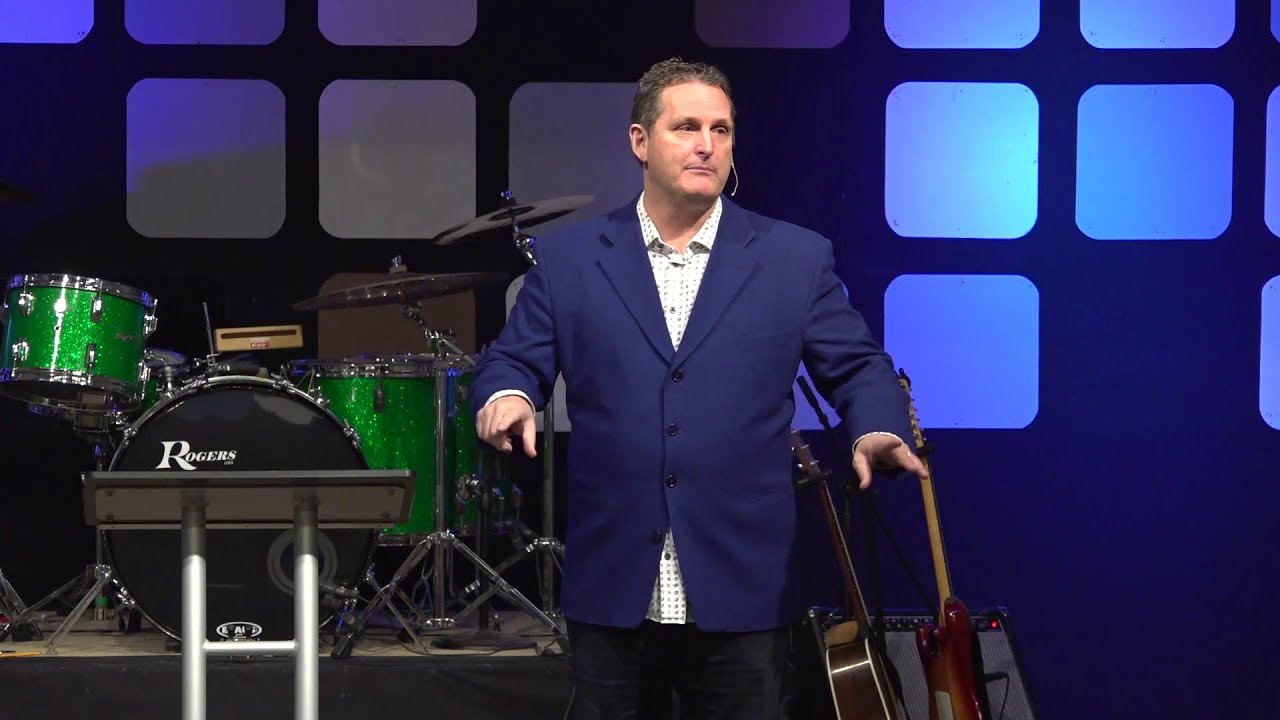The photograph depicts a slightly larger built white man in his forties, wearing a dark blue suit jacket over a white button-down shirt with a subtle black dot pattern. He has short brownish-black hair and his head is tilted to the right, with a thin microphone extending from his ear towards his mouth. His arms are raised slightly to his sides, as he appears to be addressing the audience and pointing towards a podium in front of a green drum kit on his left. The drum kit features a black bass drum with the brand name "Rogers" inscribed in white font. On his right, several guitars are stacked or leaning against an amplifier. The stage's backdrop consists of a dark blue background adorned with a pattern of light blue squares, some partially obscured, creating a mosaic-like effect.